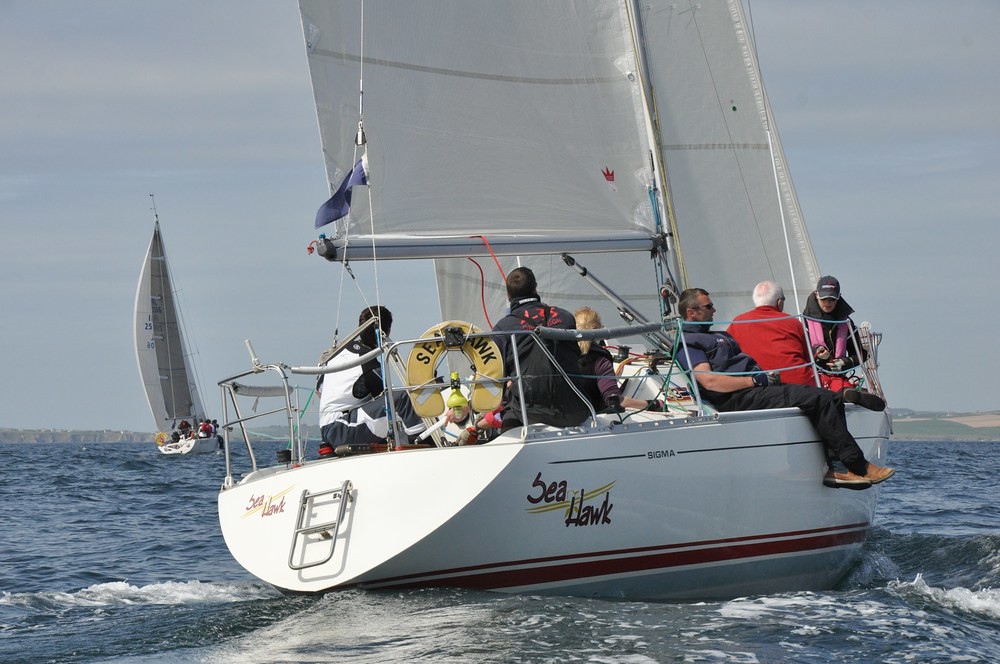In this image, we observe a white sailboat named Seahawk, viewed from the rear at an angle. The boat is crowded with many large people on the deck, with one individual notably hanging over the edge. The passengers include one person in a red shirt and another in a black shirt. The Seahawk is equipped with fencing around the deck, with visible gray-colored wires. Part of the sails can be seen at the bottom of the boat. The water around the boat displays light white caps and waves that appear bubbly against the blue ocean water. In the background, there is another white sailboat with a slightly tilted position, suggesting it might be struggling. The gray sky creates a somber atmosphere, with land faintly visible on the distant horizon.